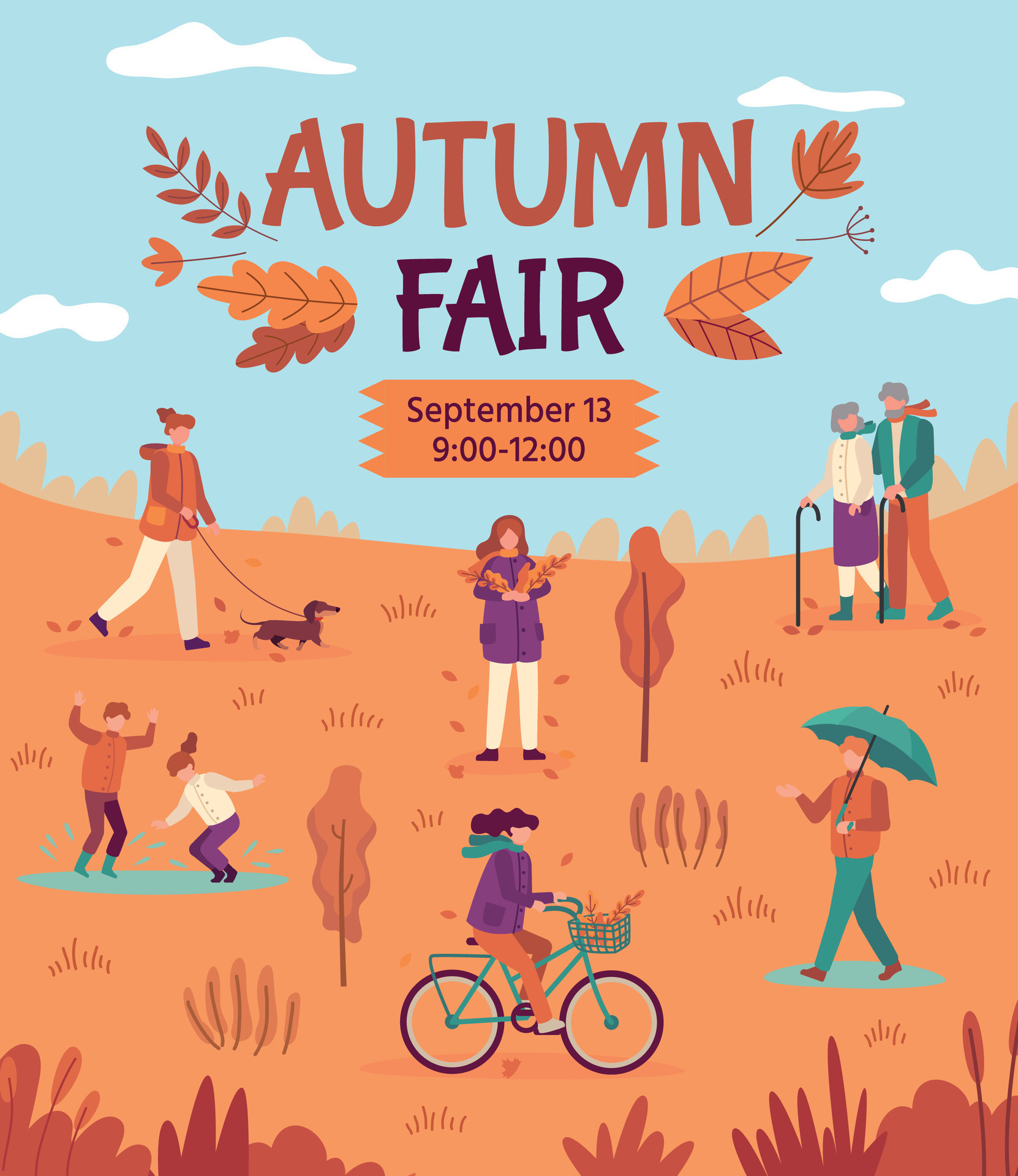The image is a detailed, computerized poster announcing an Autumn Fair. At the top, the words "Autumn" and "Fair" are written in shades of brown, flanked by orange and brown leaves. Below this title, an orange rectangle with pointed ends displays the date "September 13th" and the time "9 o'clock to 12 o'clock."

The background features a light brown, slightly yellow field dotted with darker brown weeds and plants. The sky is a blue gradient with white clouds, and orange trees grow between the horizon and the sky. 

Various people populate the scene, each depicted without faces. On the left, a woman in a brown coat, yellow or white pants, and purple shoes walks a brown and lighter brown wiener dog on a red leash. Below her, two kids play in a blue puddle; the child on the left wears a brown coat, purple pants, and blue shoes, while the child on the right is dressed in a white shirt, purple pants, and black shoes.

In the middle, a woman in a purple jacket, white pants, and black shoes carries two brown leaves. Another woman rides a blue bike, wearing a blue scarf, a purple coat, and brown pants, with brown leaves in her bike's blue basket. 

On the top right, two elderly people with gray hair walk together. One wears a white shirt, purple skirt, and white pants with a blue scarf and blue shoes while holding a black cane. The other is dressed in a bluish coat with green sleeves, a green undershirt, brown pants, and green shoes, and also uses a black cane. Below them, a person holds a blue umbrella with a black handle, dressed in an orange coat, green or blue pants, and black shoes, and walks through a blue puddle.

The landscape is completed by the presence of various green, blue, purple, and brown colors, creating a vibrant autumnal scene with the community enjoying outdoor activities.